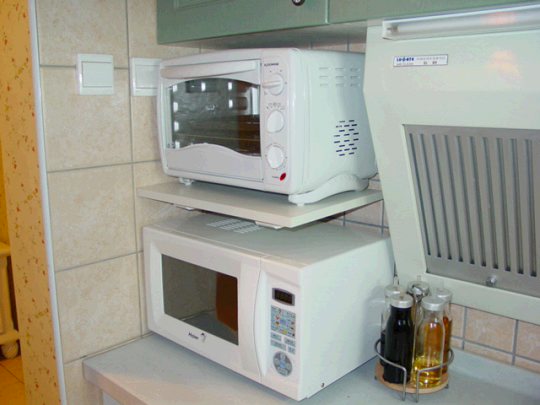The image depicts a section of a kitchen showcasing the clean and organized arrangement of white kitchen appliances and a well-stocked condiment storage. At the top, resting on a clean white surface, is a white toaster oven equipped with three knobs and a pull-down door, indicative of its pristine condition. Below the toaster oven sits a similarly clean white microwave with a digital display and gray buttons accented with red, yellow, and blue tones. The kitchen wall features a blush pink subway tile backsplash with gray grout, flanked by beige tiles and a hint of wood grain towards the left side. To the right of the microwave, beneath a closed vent hood, stands a lazy Susan displaying various bottles of oil, vinegar, and other liquid condiments. The well-lit and neatly arranged kitchen evokes a modern European aesthetic.